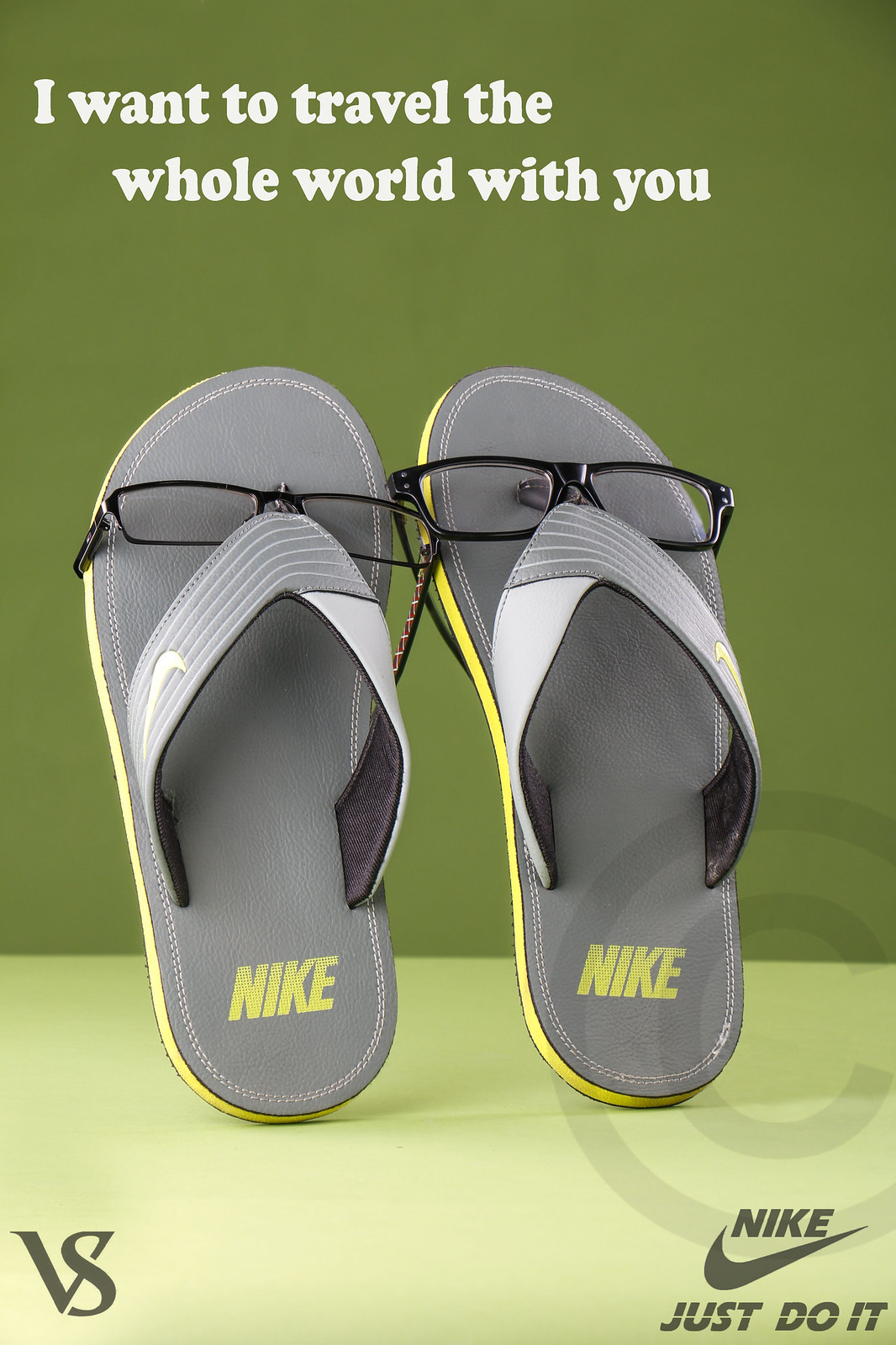This is an advertisement for Nike flip-flops that seems to be designed for a magazine spread. The image prominently features two pairs of light gray Nike flip-flops with yellow accents, including the Nike swoosh logo on the side straps and the word "Nike" written at the base of the footbed. Notably, the flip-flops also have black-framed glasses resting on them, adding a whimsical touch. The flip-flops are set against a green background, with the upper portion of the backdrop being a medium green and transitioning to light green at the bottom. At the top of the image, in white text, is the phrase, "I want to travel the world, the whole world with you." The bottom-right corner showcases the Nike logo along with the famous slogan "Just Do It," while the bottom-left corner displays a "VS" logo. The overall composition emphasizes a travel theme intertwined with the casual, sporty style of Nike flip-flops.